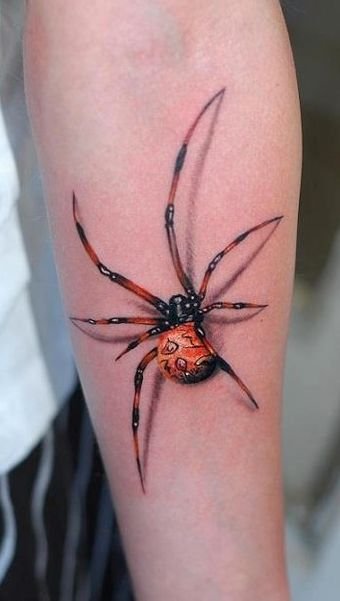In the photograph, the main focus is a large spider resting on a white person's left forearm, extending from the wrist to the elbow, seen from the upper side showing the bend of the elbow. The individual's arm appears slightly reddened where the spider sits, though they seem unbothered, merely allowing the spider to crawl on their skin. The person is dressed in a white shirt and black pants with white vertical stripes, visible in the left portion of the image. The spider is notable for its imposing size, with legs that are extremely long and slender, almost half the length of the forearm, and are a combination of light red and black. The spider's body is round, large, and predominantly light red with almost diamond-shaped black outlined patterns. Its head is entirely black, and the legs are hairless, adding to the striking appearance of this arachnid.